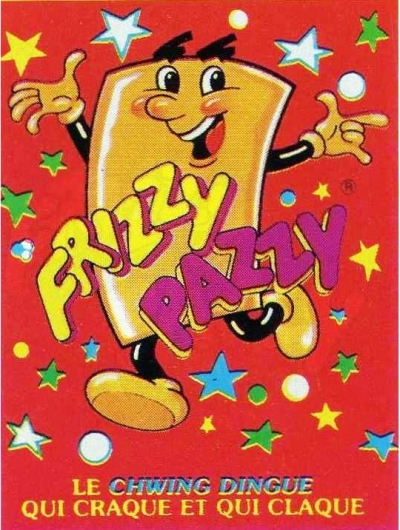The image depicts a smiling yellow cylindrical cartoon character with white reflections on its sides, running to the left against a red background. The character has thin black limbs, wears yellow gloves and boots, and raises both hands in the air. The character’s face features eyebrows above its head and a mouth open in a jovial expression with a visible red tongue. Surrounding the character are colorful stars and dots in hues of green, blue, white, and yellow. Above the character, bold text reads "Frizzy Pazzy," with "Frizzy" in yellow and "Pazzy" in purple. At the bottom of the image, there is French text in all capitalized letters saying "LE CHWING DINGUE" in blue, followed by "QUI CLAQUE ET QUI CRAQUE" in yellow.